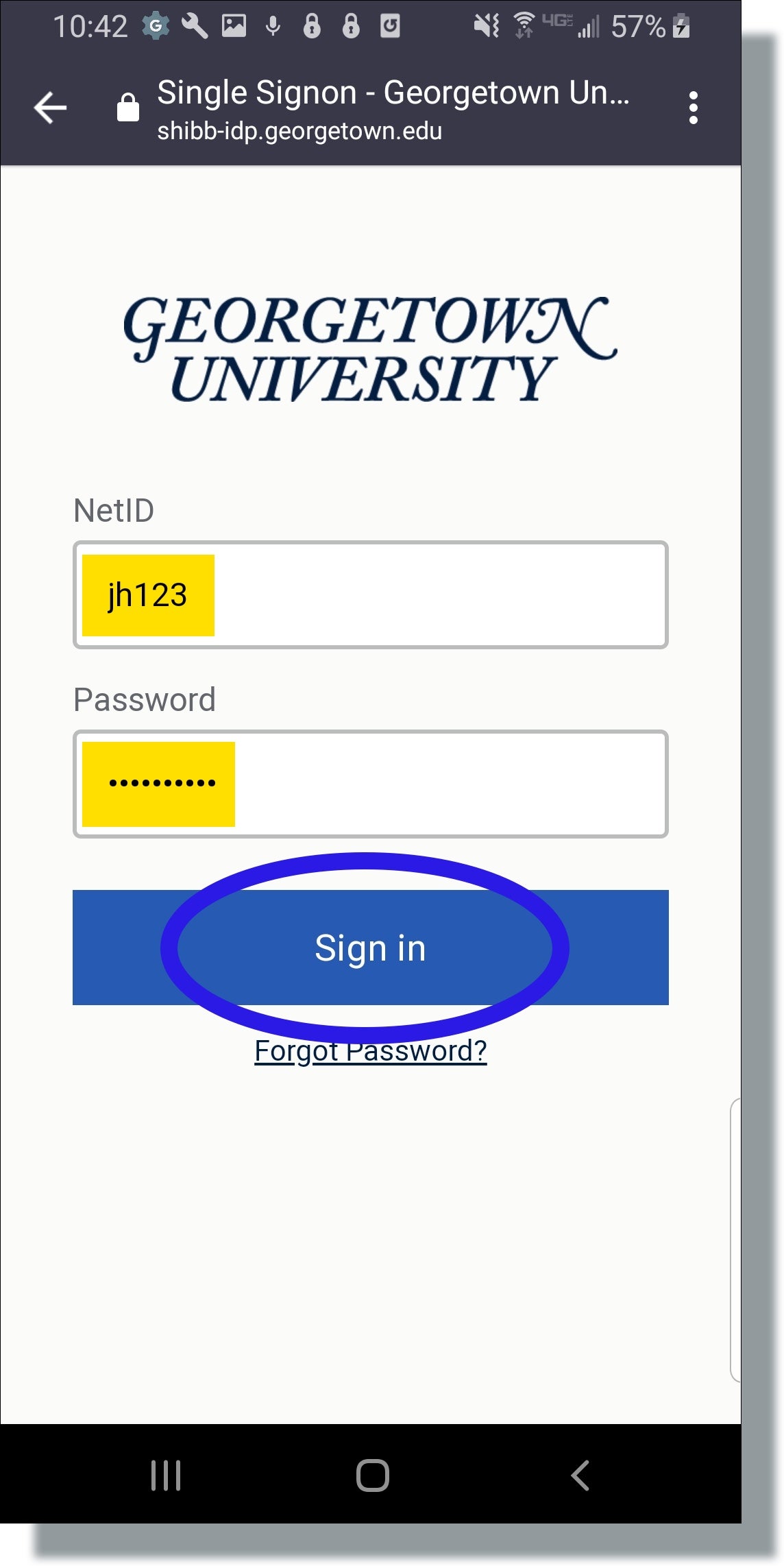This image is a cropped screenshot of the mobile login interface for the Georgetown University website. The background is predominantly white, focusing attention on the central elements. At the top, "Georgetown University" is prominently displayed in large blue font. Positioned below are two text boxes.

The first box, labeled "NetID" in grey text at the top left, has "JH123" typed within it, highlighted with a yellow overlay to emphasize the placeholder text. Directly beneath, the second box is labeled "Password," also in grey text at the top left. Inside, the password is obscured by dots, and this box too is highlighted in yellow.

At the bottom of the screenshot, a blue "Sign In" button is prominently featured. A blue oval has been added to the image, encircling the button, further emphasizing the next action step. This instructional screenshot visually guides the user through the login process, indicating the need to enter their NetID and password before clicking the "Sign In" button.